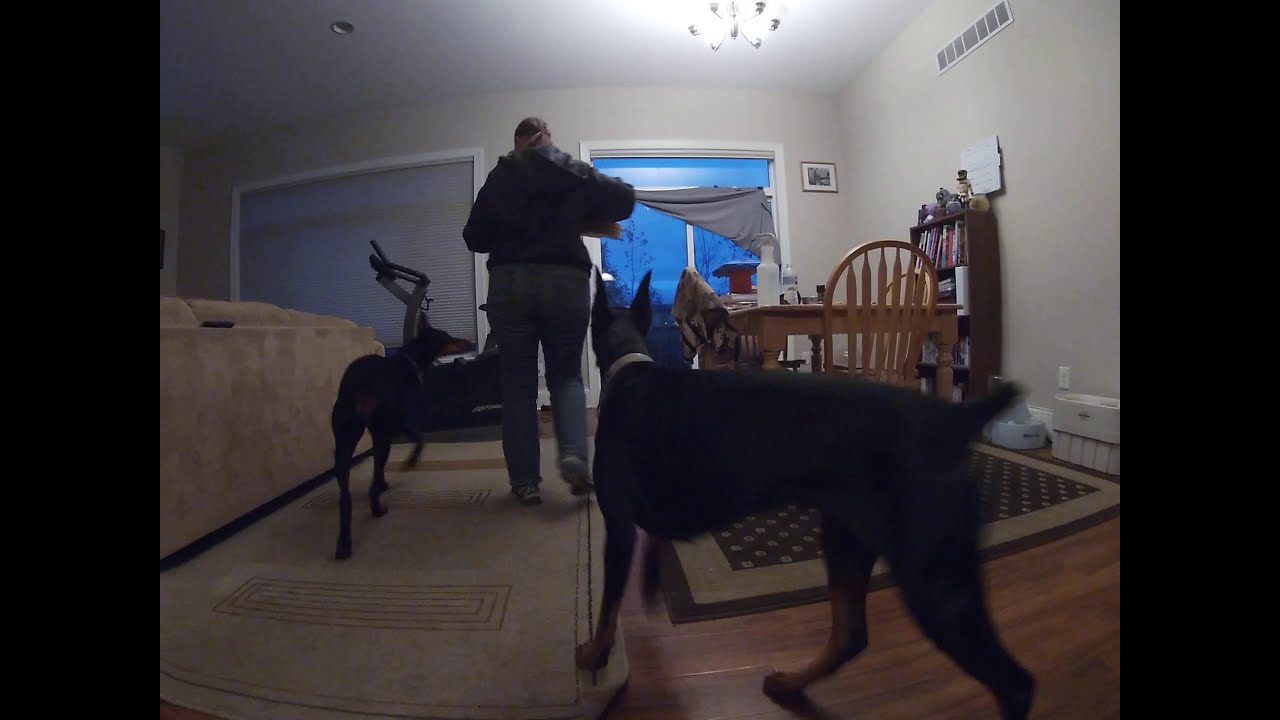The image captures the inside of a house, divided into a living room on the left and a dining room on the right. The walls are white, paired with a white ceiling. The living room features a cream-colored sofa backed against a sliding glass door on the right and a large window on the left. In the center of the image, a woman with dark hair in a ponytail, dressed in jeans, tennis shoes, and a blue hoodie, walks towards the sliding glass door, accompanied by two large black Dobermans with distinctively pointy ears, one on her left and the other a few steps behind.

The dining room showcases a small, rectangular wooden table with four wooden chairs, situated on a brown and black rug. Under this rug, there's hardwood flooring, contrasting with a separate tan carpet seen on the living room side. To the right of the dining table, a small wooden shelf holds various items, including books and some indistinguishable articles. Near the shelf, there's what appears to be a dog water bowl. The background features both the sliding glass door and the large window, both contributing to the room's inviting natural light.